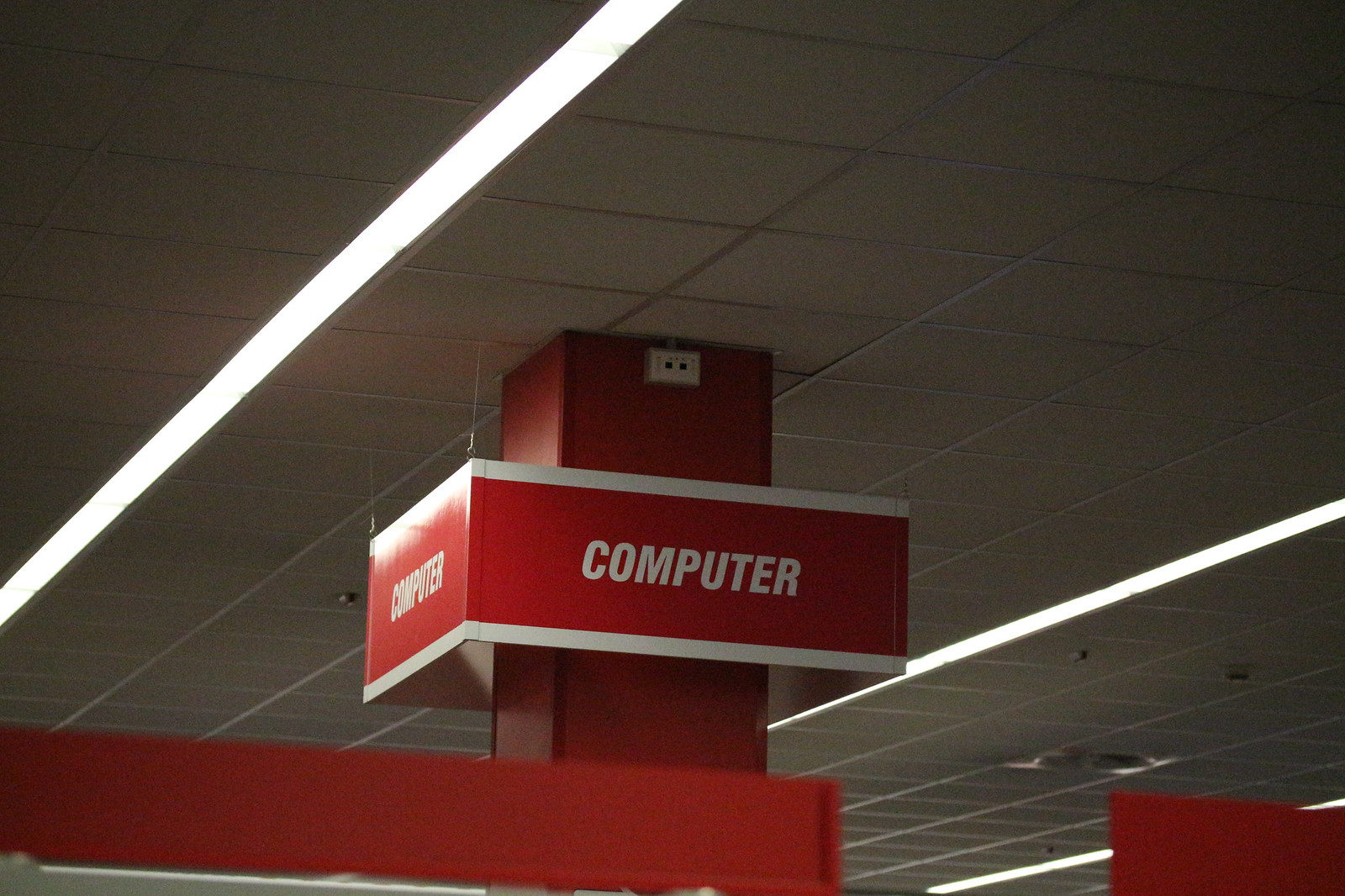The photograph captures an interior shot of a store. The ceiling, composed of a grid of square tiles, forms the backdrop at the top of the image. Illuminating the space are long, linear light fixtures extending from the left towards the right and the bottom right, receding into the background.

In the center of the image, an imposing red beam descends from the ceiling. Attached at its top is a white box, likely a power outlet or plug-in. Further down the beam, a circular red banner with white stripes wraps around. Adorned with large white letters, the banner prominently displays the word "COMPUTER" on all visible sides.

At the very bottom of the image, a red, rectangular canopy appears, which seems to be the top part of a shelving unit, adding structure to the framed scene.